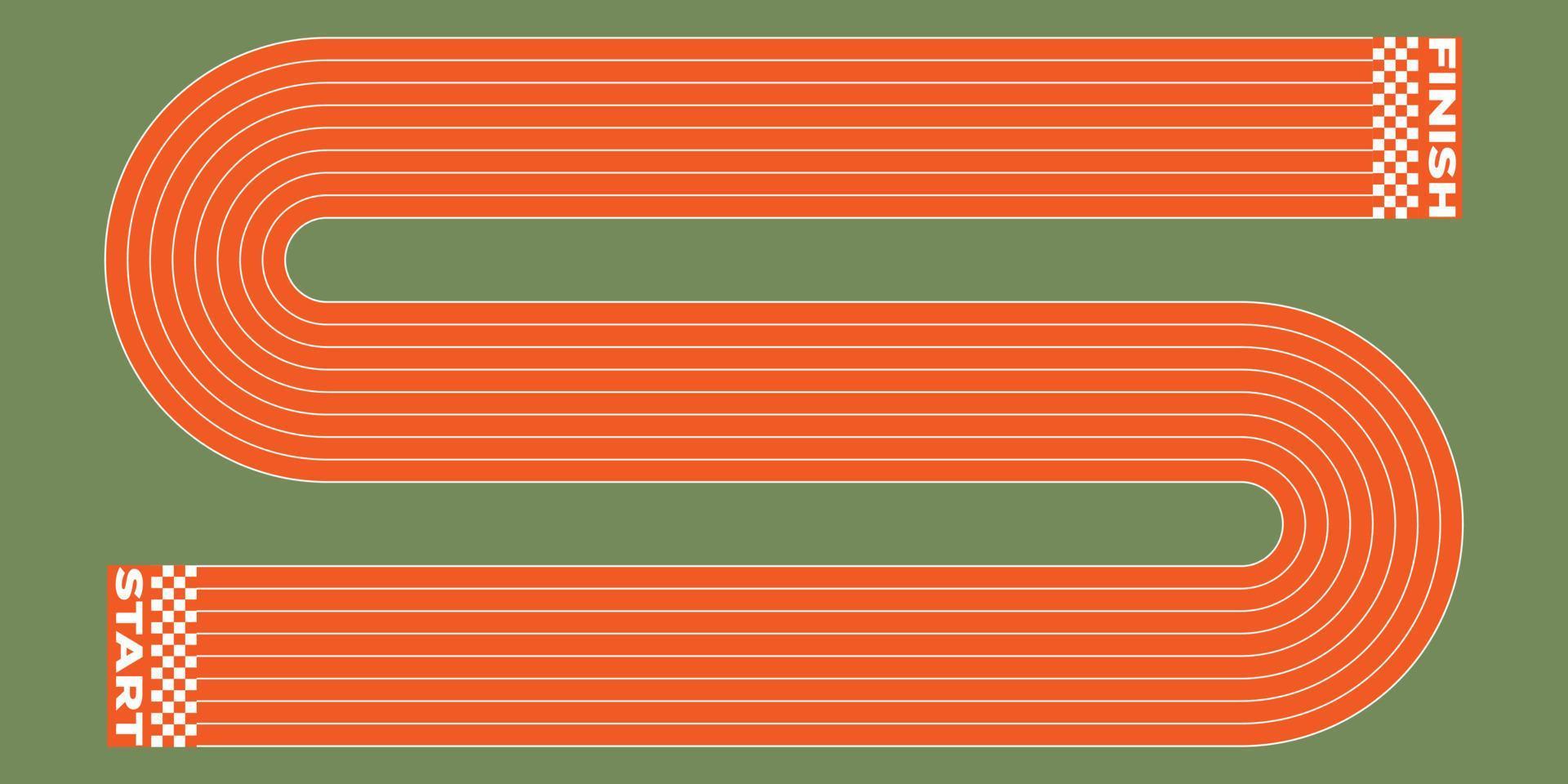In this image, a graphic design or possibly a logo, features a bird's eye view of an orange racetrack set against a brownish green rectangular background. The racetrack is depicted in an S shape with two distinct curves. Starting at the bottom left corner, where "START" is written in white capital letters accompanied by a traditional starting line with white lane stripes, the track winds to the right, curves downward, snakes back to the left, and curves again downward before reaching the top right corner. Here, "FINISH" is written vertically in white letters along a checkered finish line. The track comprises eight lanes, clearly marked by white lines that run the length of the course.